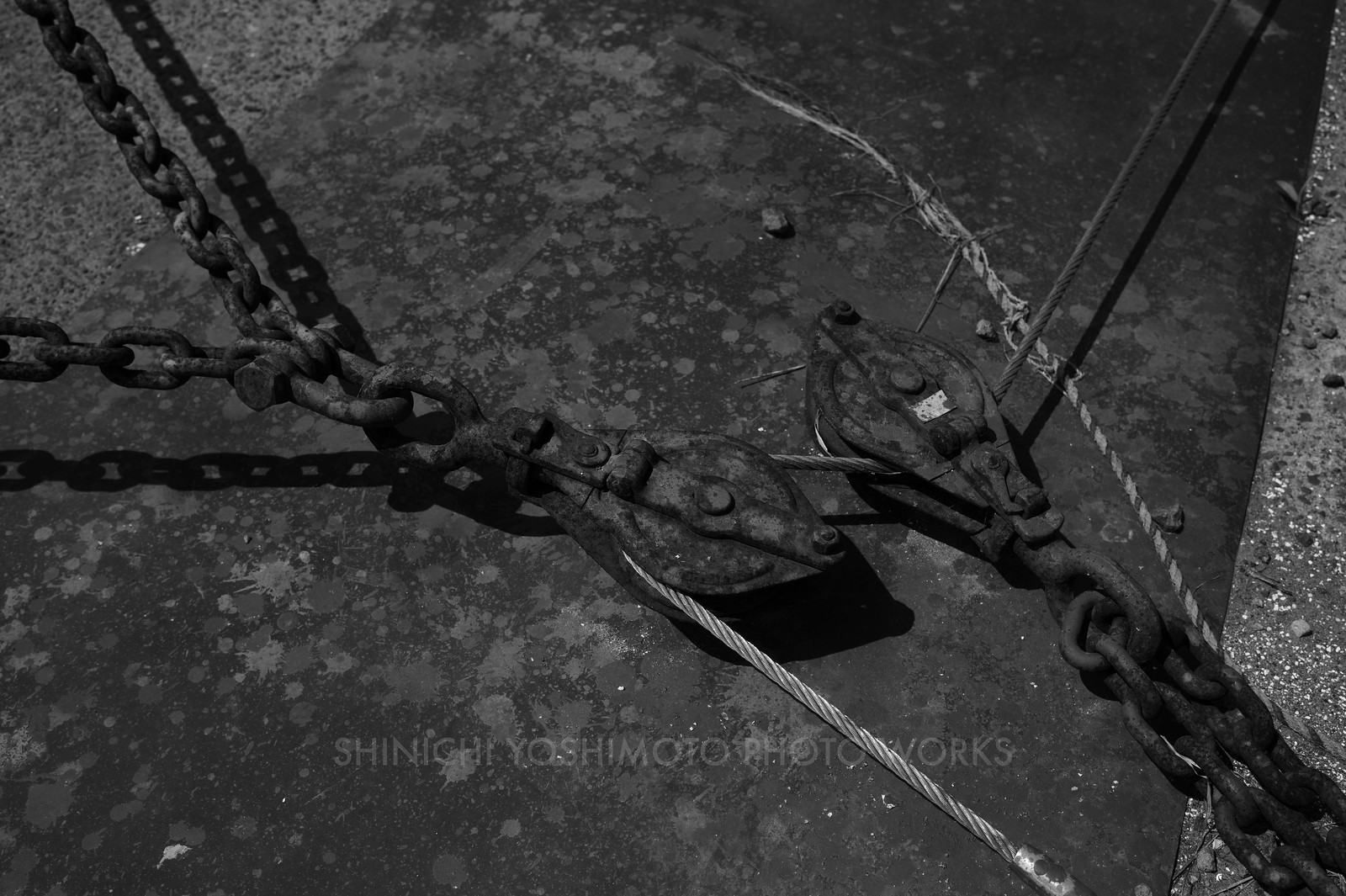This black-and-white photograph, titled "Shing-Hee Yoshimoto Photo Works," captures a detailed close-up of a complex chain and pulley system. The composition, in landscape orientation, features two heavy chains that converge at the center, where they are interconnected by a braided rope. This rope weaves through two pulleys positioned in the middle of the frame, then extends off the image to the upper right and lower right corners. The pulleys are held by hooks connected to additional chains that spread out in a V-shape on either side. The background of the image consists of what appears to be a large steel plate, contrasting with the dark metal chains and rope. The chains also appear to lie atop a metal structure underneath, adding more texture and depth to the industrial scene. Beneath this meticulously arranged mechanism, a line of light white text reads "Shing-Hee Yoshimoto Photo Works," distinguishing the piece with artistic authenticity.